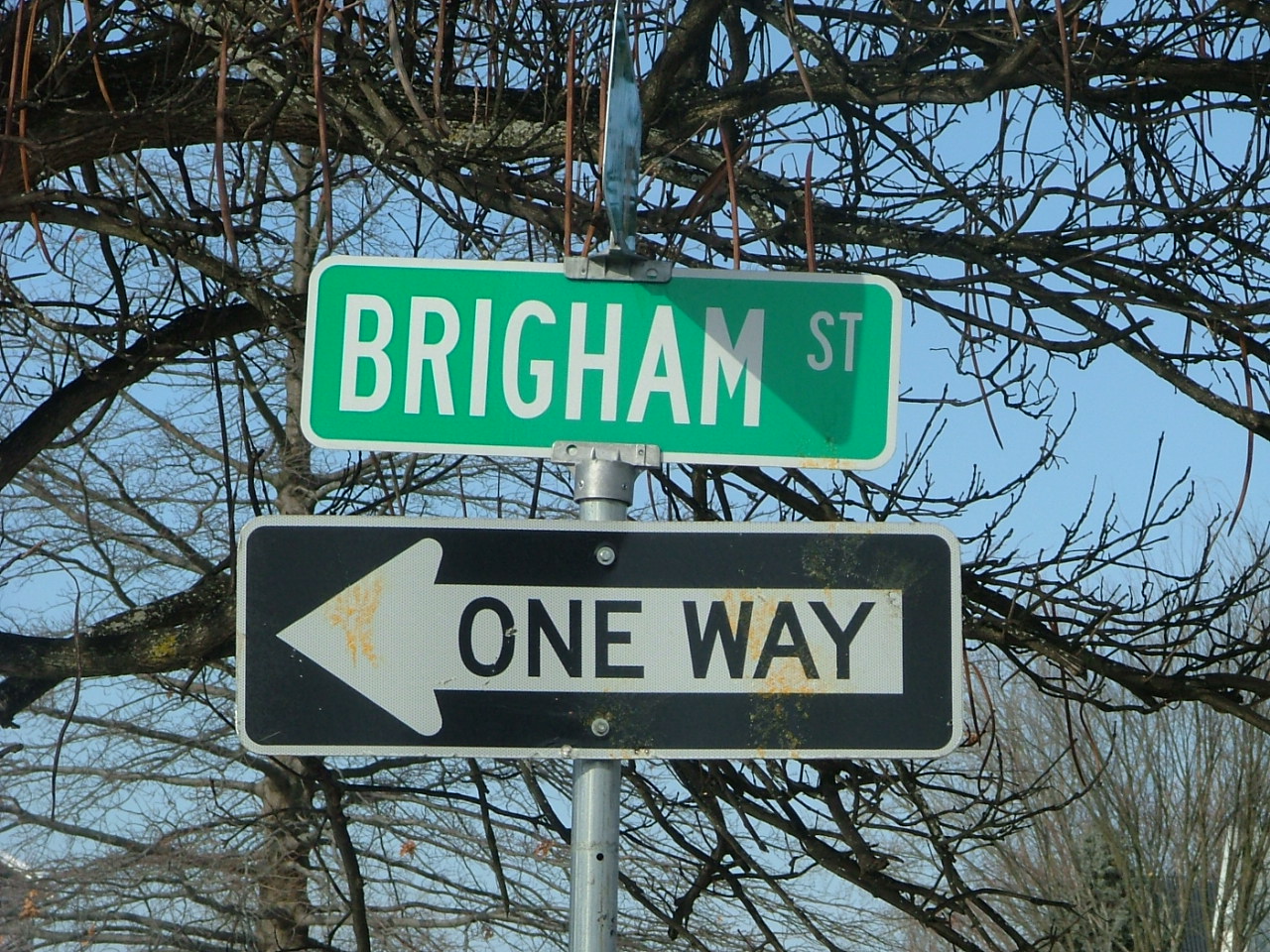In this daytime photograph, two street signs are prominently displayed against a clear, blue sky. The background features leafless trees, adding a stark yet serene ambiance. The top sign is a rectangular, green street sign reading "Brigham Street," while the lower sign is a white-bordered, rectangular one-way sign, boldly indicating "One Way" with an arrow pointing to the left. The image captures the quiet, almost minimalist beauty of an urban landscape in late fall or winter.